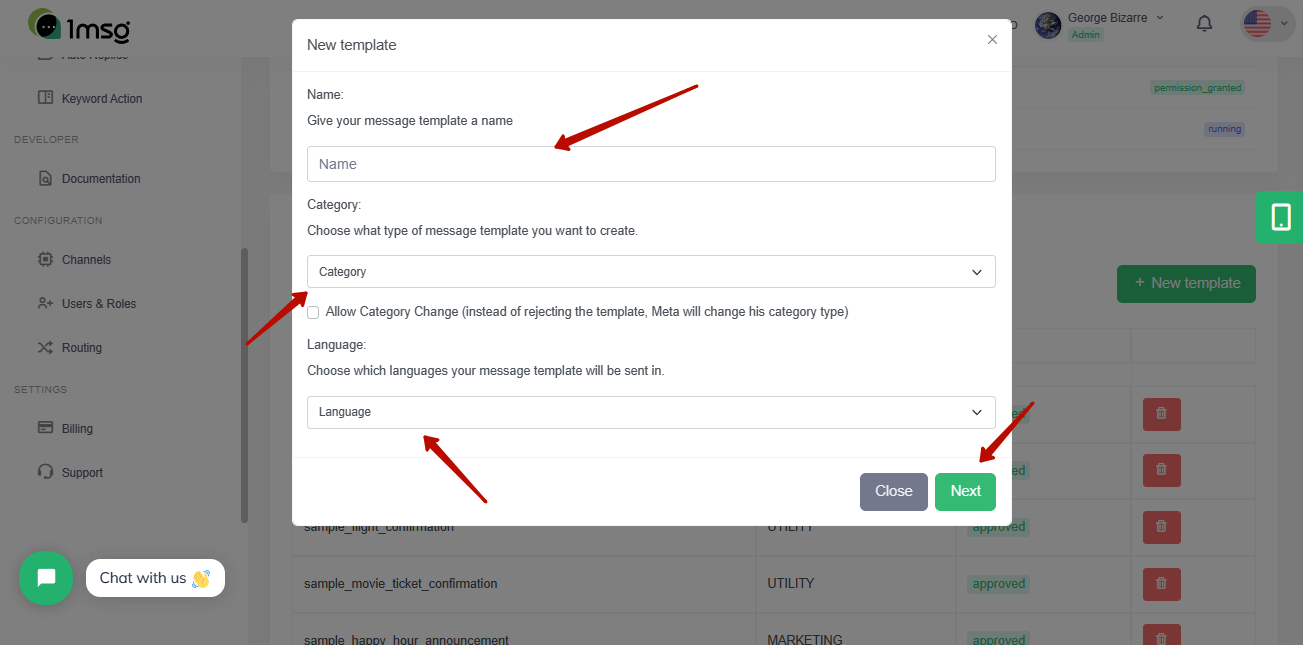This image showcases a screenshot from a website or platform named "1Message," stylized peculiarly as "1MSaG." The logo features a stylized "G," with a circle representing its upper part, a small curved line beneath it, and a dot above the circle, giving it an unusual appearance.

At the center of the image is a pop-up box titled "New Template," indicating that the user is on a screen where they can create a new message template. The first field in this pop-up is labeled "Name," accompanied by a prompt to "give your message template a name," with a textbox for input. Below this is the "Category" section, instructing the user to choose a type of message template from a drop-down menu of categories.

Further down, there's an unchecked checkbox labeled "Allow category change," with an explanation that instead of rejecting the template, Meta will change its category type if needed. This is followed by a "Language" field, where users can select the language(s) in which their message template will be sent from another drop-down menu.

At the bottom of the pop-up, there are two buttons: a "Close" button on the left and a "Next" button on the right, allowing the user to either exit the screen or proceed to the next step in the template creation process.